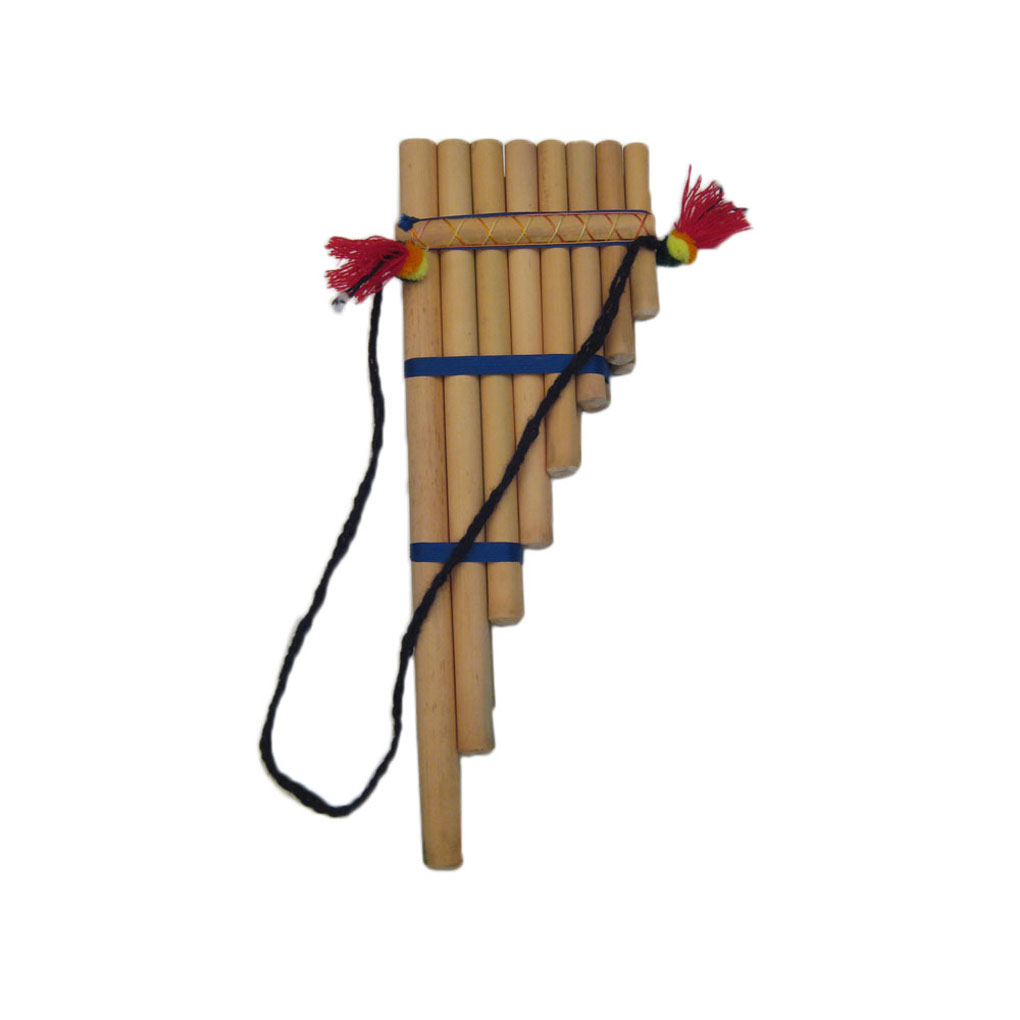The image displays a finely crafted wooden pan flute set against a white background. This traditional wind instrument, designed to produce melodious notes when blown into, features approximately eight wooden pipes arranged in decreasing length from left to right. The pan flute is bound together with intricately placed colored ribbons: the three longest pipes are tied with blue ribbon; an additional set of three pipes is secured with red ribbon; and all pipes are collectively bound at the top with a blue and brown ribbon embossed with brown X's. Attached to this top ribbon is a black rope intertwined with red, yellow, and black knots, serving as a strap for easy handling or wearing around the neck. The instrument's elegant brown wooden texture, enhanced by the vibrant ribbon colors, highlights its traditional aesthetic and craftsmanship.